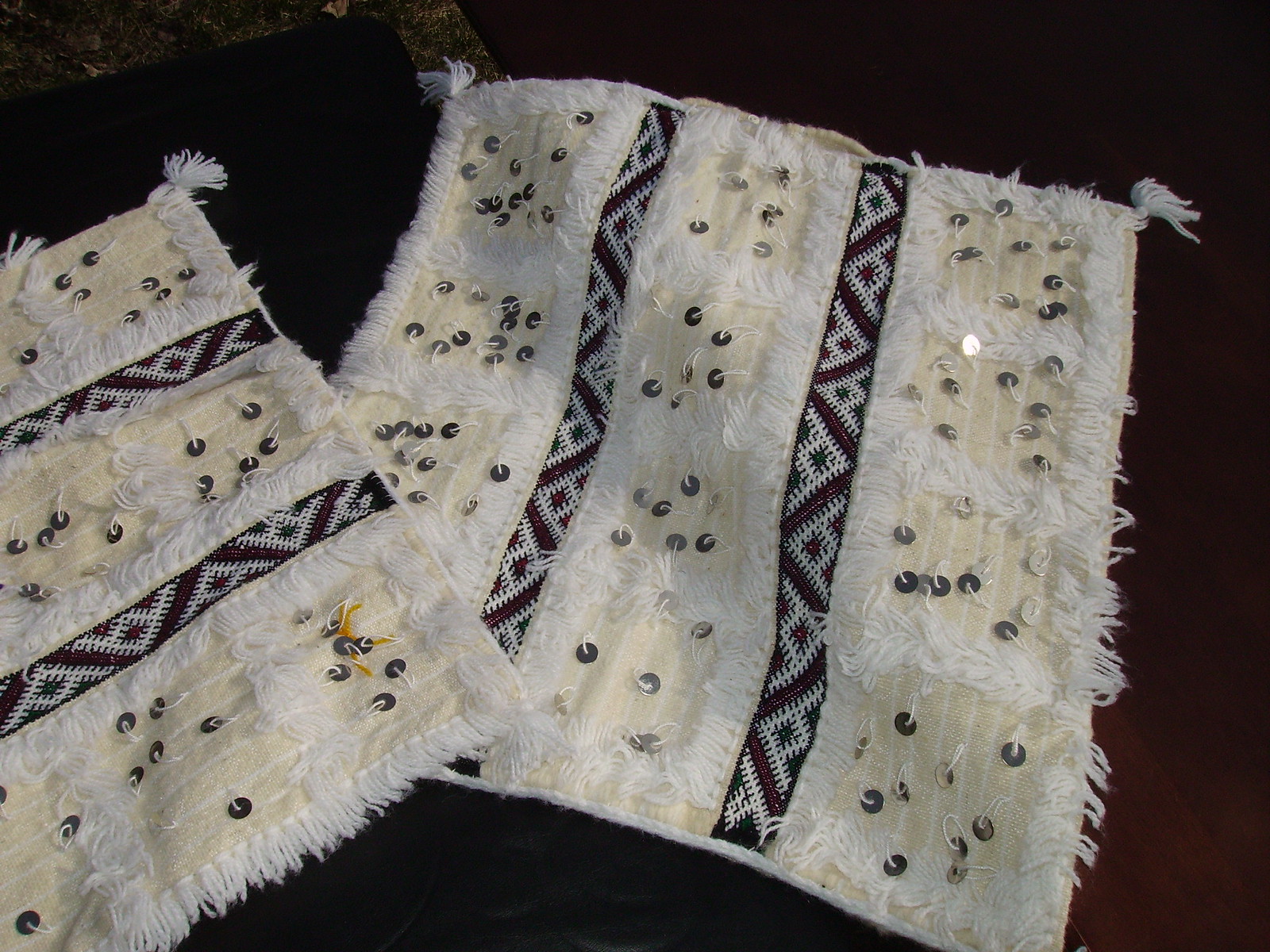This image showcases a pair of intricately designed fabric pieces, likely decorative quilts or small blankets, arranged on a dark, indistinct surface. The quilts feature a striking zigzag and squiggly pattern in shades of brown and white, giving them an appearance reminiscent of an Indian print. Each quilt is adorned with beads, dark sequins, and buttons, adding a touch of shimmer and texture. The edges are finished with light beige and white fringes. The layout of the designs includes two central median strips with intermittent patterned patches, making these items not only functional but also visually captivating. The photograph is taken in a dimly lit setting, highlighting the contrasting colors and intricate details of the fabrics against the dark backdrop.